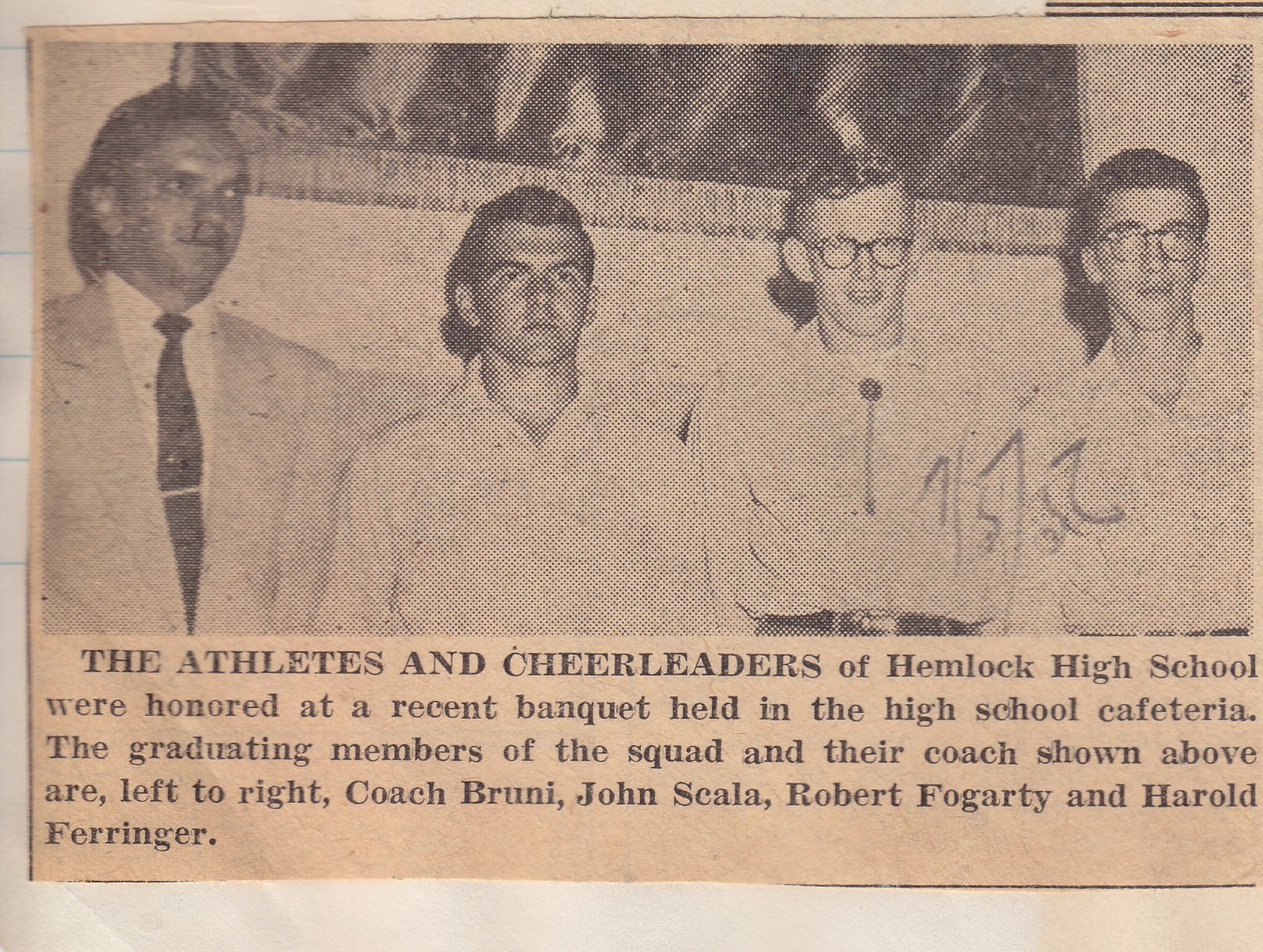This vintage newspaper clipping, with a sepia-toned, peach-colored paper, features a black and white photograph of four men standing side-by-side, identified as the graduating members and coach of the Hemlock High School squad. The caption beneath the photo reads: "The athletes and cheerleaders of Hemlock High School were honored at a recent banquet held in the high school cafeteria. The graduating members of the squad and their coach, shown above, are, from left to right, Coach Bruni, John Scala, Robert Fogarty, and Harold Barringer." The older gentleman on the left, Coach Bruni, is dressed in a jacket and tie, exuding a formal demeanor. To his right, John Scala stands with a serious expression, wearing a finely groomed look and a buttoned white collar shirt. Robert Fogarty and Harold Barringer, also in white long-sleeve shirts, complete the group. In the background, a wall bearing part of a banner, likely clipped by the photograph, hints at the celebratory setting of the high school cafeteria where the banquet took place. The image, appearing to date from the 1950s or 60s, exudes a nostalgic charm.